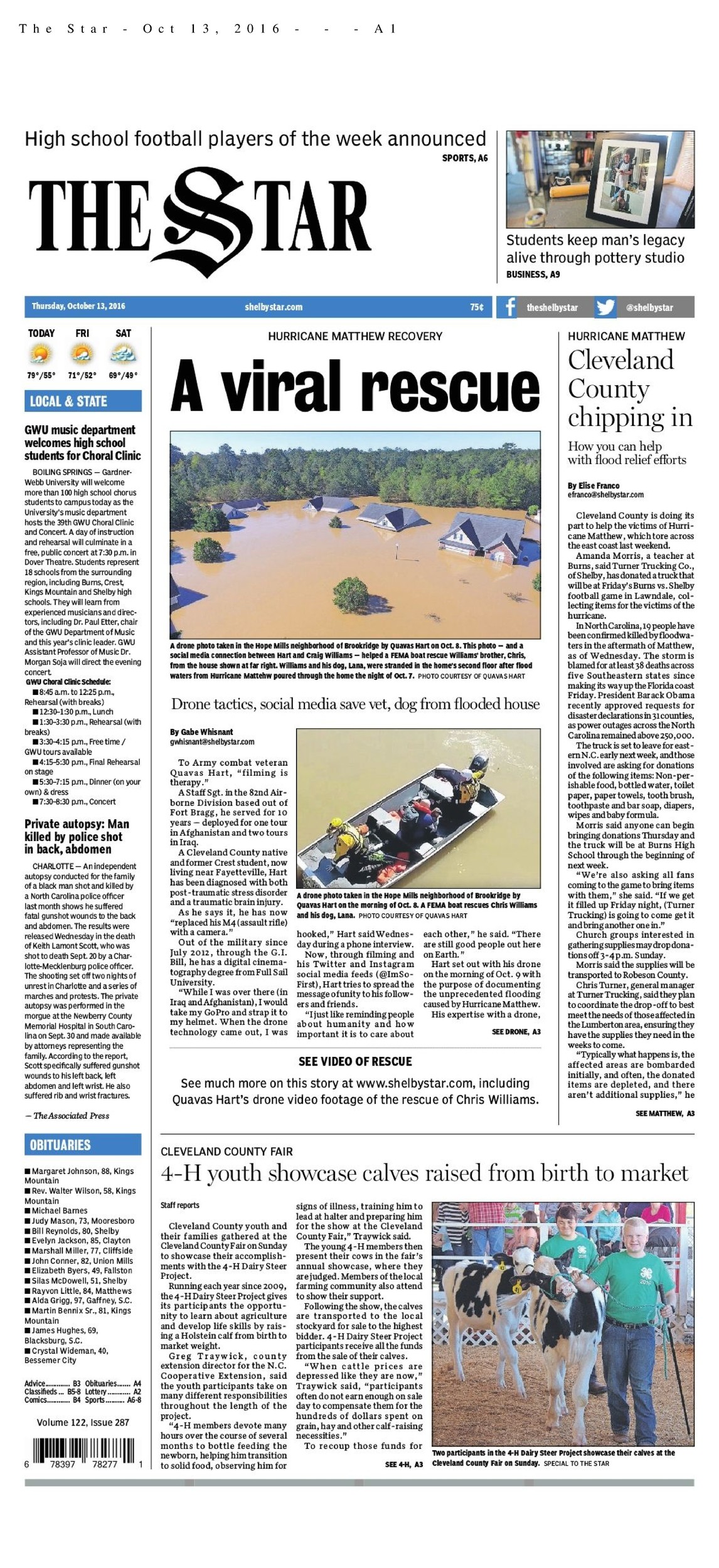The image depicts the front page of a newspaper, presenting a classic monochromatic layout with black text on a white background, accented by blue labels highlighting specific sections. The masthead at the very top reads "High School Football Players of the Week Announced on Sports A6." To the immediate right, another headline proclaims, "Students Keep Man's Legacy Alive Through Poetry Studio Business A5 or A9," though the precise page number is somewhat unclear.

Beneath this, a prominent black star graphic is noticeable. On the upper left portion of the paper, the current weather information is displayed. Furthermore, a notable headline titled "A Viral Rescue" catches the eye. Accompanying this is an article elaborating on "Drone Tactics, Social Media Save Vet's Dog from Flooded House."

Another significant headline on the page reads, "Private Autopsy: Man Killed by Police Shot in Back and Abdomen," indicating a serious investigative piece. At the bottom of the page, an article titled "4-H Youth Showcase Calves Raised from Birth to Market" covers a feature on agricultural youth programs. Lastly, in the top right corner, a community story is highlighted with the headline, "Cleveland County Chipping In for Hurricane Matthew."